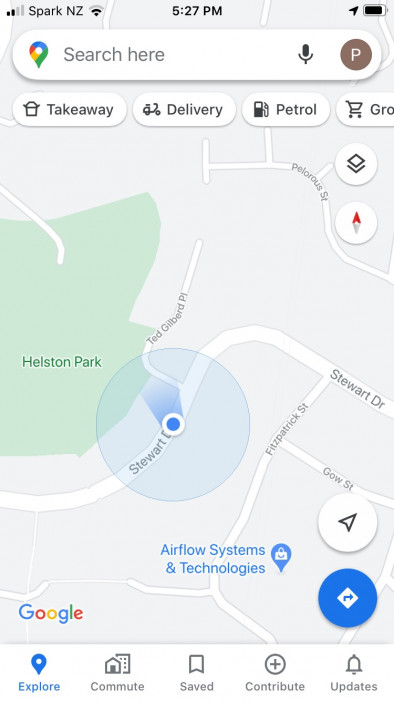This image showcases a smartphone displaying a map. At the top of the screen, it indicates the network provider, "Sparks NZ". The battery life icon shows approximately 95% charge, and the current time is 5:27. Just below the top bar, there is a search bar marked by a multicolored Google Maps pin icon, prompting "Search here." On the right side of the search bar, there is a microphone icon and a brown circle with the letter "P" within it.

Underneath the search bar, there are quick-access tabs labeled "Takeaway," "Delivery," "Petrol," and "Groceries." The map also highlights specific locations: "Hyaston Park" is prominently shown in green, and nearby is "Airflow Systems and Technologies," marked in blue. Additionally, a blue dot with radiating lines—representing the user's current location—is situated near "Stewart Drive," although the "DR" abbreviation is partially obscured. The bottom of the screen features a "Directions" button on the right and the word "Google" on the left.